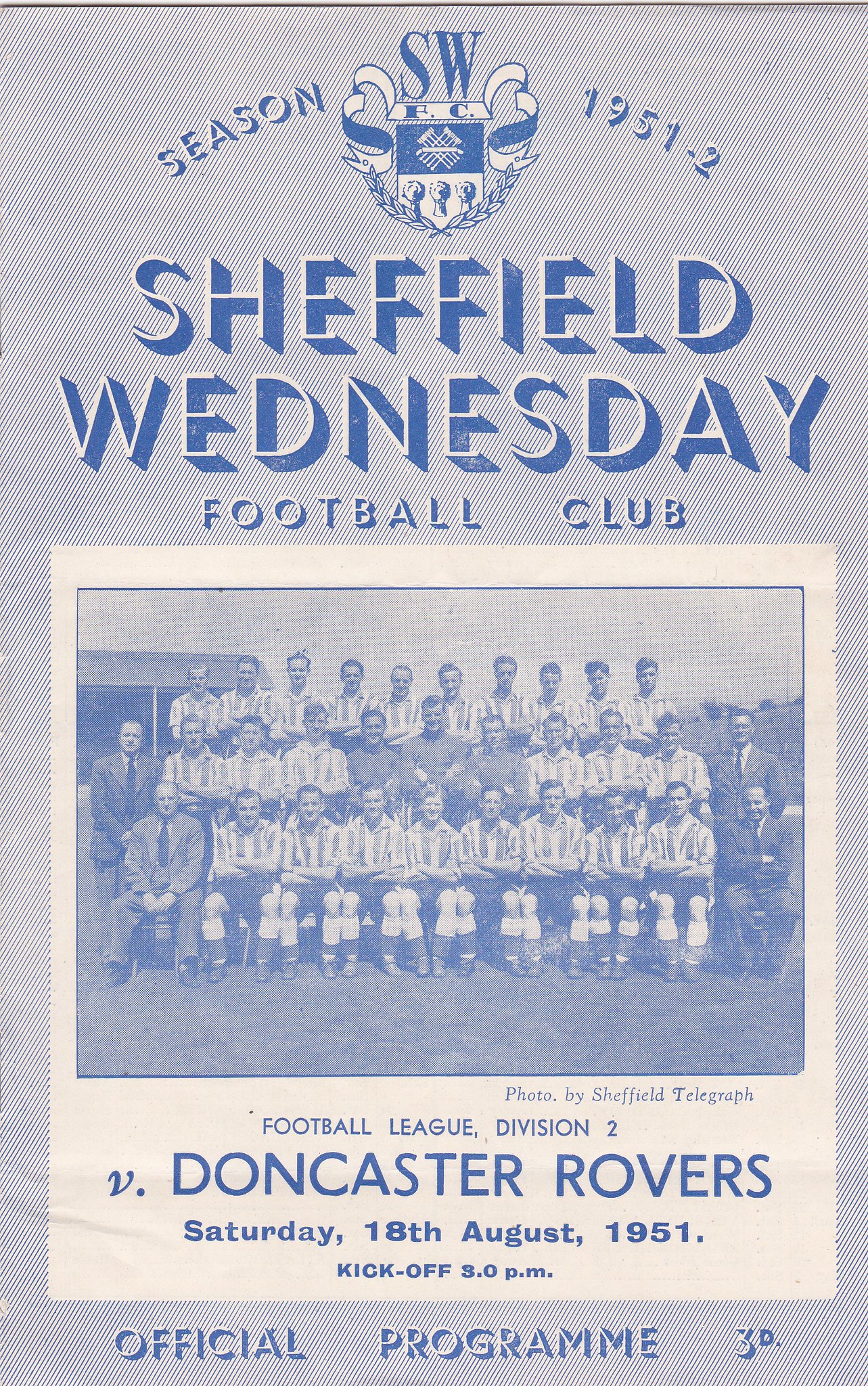This image is the cover of an official program for a football match from the 1951-52 season, featuring a detailed blue and white design. Prominently displayed is the Sheffield Wednesday Football Club's crest. At the top, the text reads "Season 1951-52, Sheffield Wednesday Football Club." Centered below the title is a group photograph of the team, consisting of three rows: the front row seated and the back rows standing, with coaches in suits flanking the players in uniforms. The caption notes the photo is by the Sheffield Telegraph. Below the team image, the text announces the event: "Football League, Division II, versus Doncaster Rovers, Saturday 18 August 1951, Kickoff 9 p.m." The program is marked as the official edition with a price of 3D.